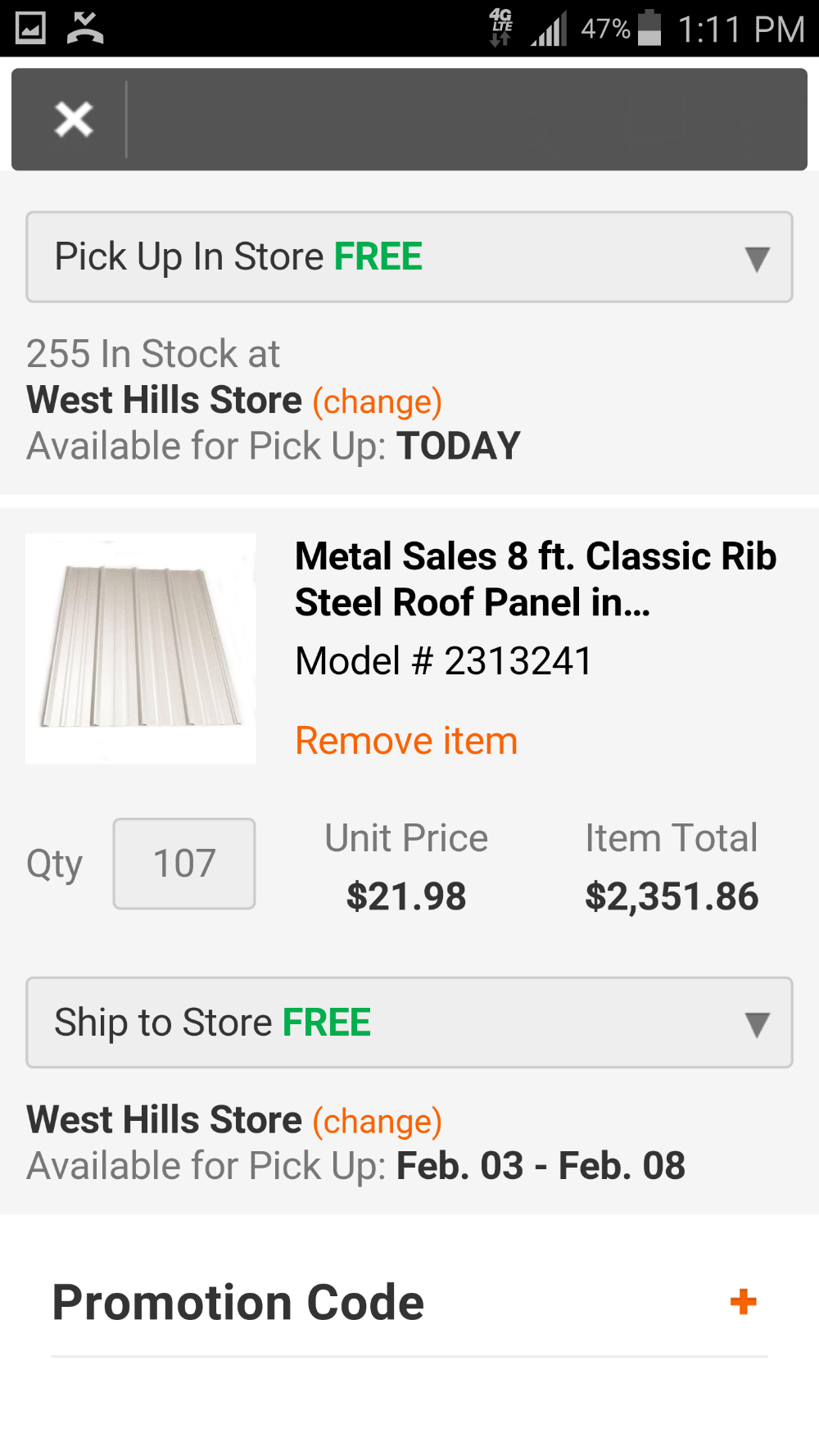The image displays a detailed screenshot of an individual order pickup entry panel on a smartphone, capturing the specifics of an item selection process. The primary focus is on a "Metal Sales 8-Foot Classic Rib Steel Roof Panel," model #2313241. The screen exhibits an image of the gray metal panel, which consists of four smaller panels joined together to form a larger unit.

On the top edge of the phone screen, typical status icons are visible: a missed call icon, a 4G network indicator showing four out of five bars, a battery level at 47%, and the current time displayed as 1:11 p.m.

The user interface reveals options for purchasing the item, with selections available for "In-store pickup" and "Ship to store," both free of charge. The "In-store pickup" option is highlighted in bright green, emphasizing its availability. It is noted that 255 items are in stock at the West Hill store, with an option to change this location presented in orange text.

Additionally, the order panel confirms that the item is available for same-day pickup, as indicated by the bold "AVAILABLE TO PICK UP TODAY" note. The user has specified a quantity of 107 units, each priced at $21.98, summing to a total of $2,351.86.

Beneath the order summary, there is a drop-down menu for selecting the store location, defaulted to the West Hill store. The availability window for this location is noted as February 3rd to February 8th. Below this, there is an option to enter a promotion code, which remains collapsed and represented by an orange plus sign button.

The overall design of the app is presented in pale gray with darker gray header banners, providing a stark yet organized contrast for ease of navigation.